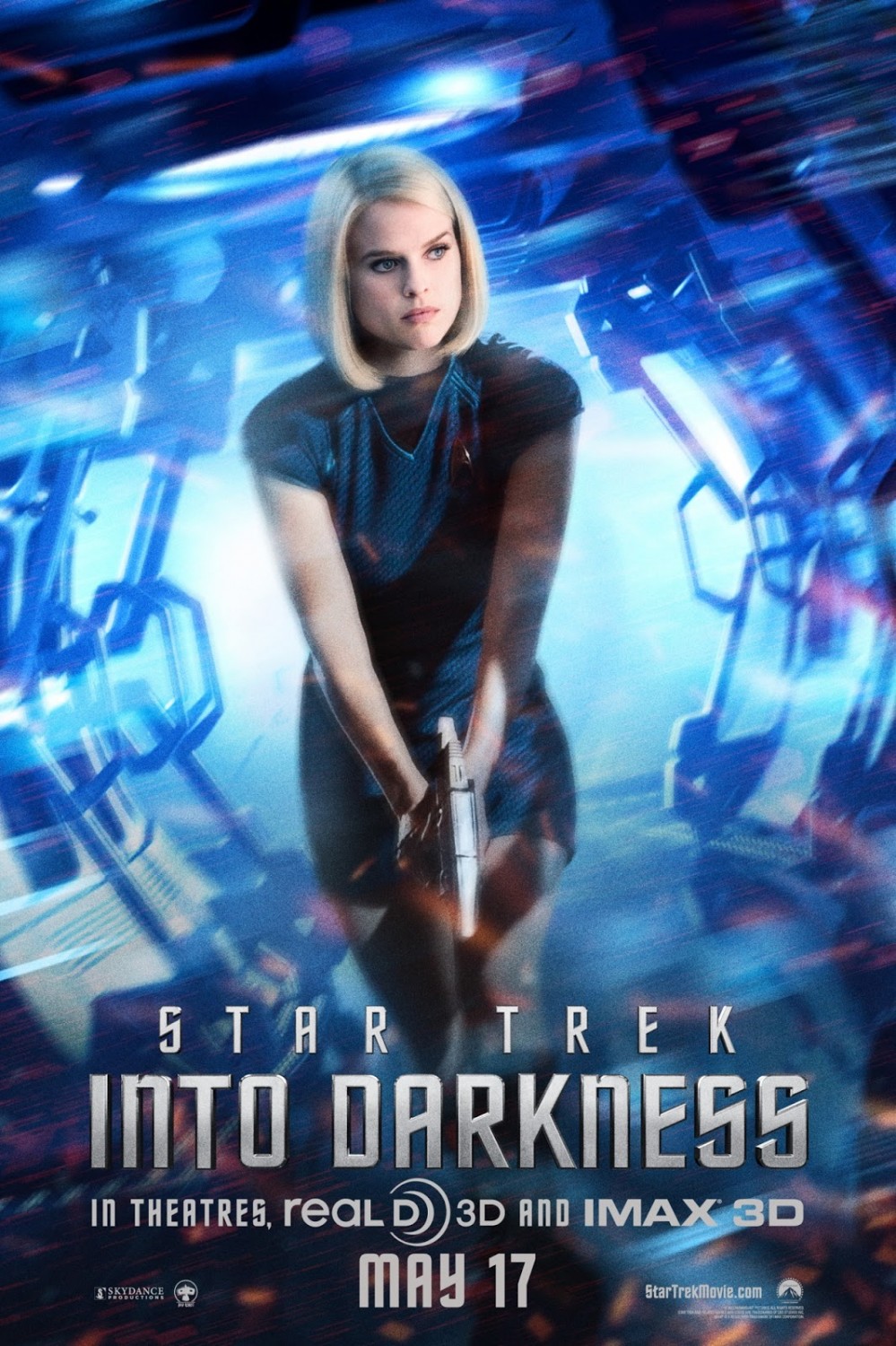The movie poster for "Star Trek Into Darkness" features a beautiful blonde woman with straight shoulder-length hair, standing prominently at the center of the image. She appears slightly distracted, looking off to her right, while holding a silver blaster in her outstretched arms. She is dressed in a dark blue, short-sleeved uniform with a short skirt. The background depicts a futuristic, hexagonal hallway with a metallic, blue, and silver color palette, illuminated by white and pink lights. The text at the bottom of the poster displays "Star Trek Into Darkness" in silver Star Trek font, with "Into Darkness" larger and more prominent. Below that, it reads, "In Theaters Real D 3D and IMAX 3D," followed by the release date "May 17th." Additional small text includes the website StarTrekMovie.com and logos for Paramount and Skydance.